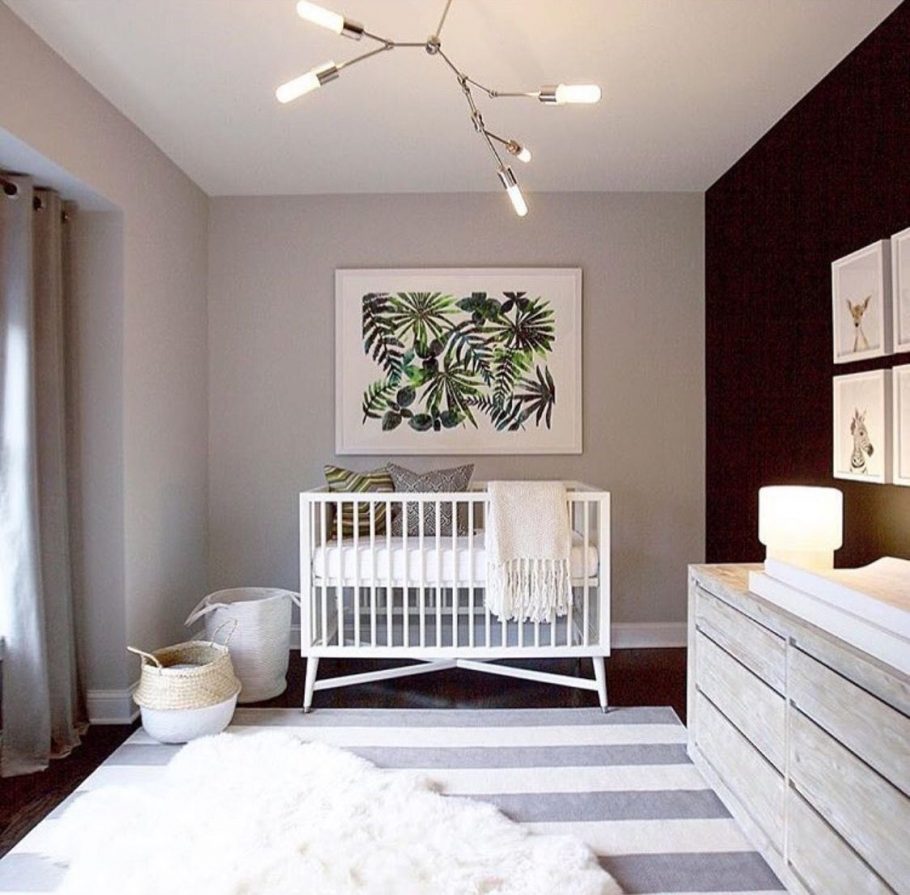The image features a room with a mix of decor styles and elements that contribute to a functional yet unadorned atmosphere, hinting at it possibly being a temporary setup such as a hotel room. Dominating the composition, the back and left side walls are grey, while the right wall is black, adding contrast to the space. A window on the left side is draped with a grey curtain, and the ceiling is illuminated by a light fixture containing four rectangular tube lights.

Central to the room is a picture hanging on the grey wall, showcasing green plants, adding a touch of nature. Below this artwork is a white baby crib, fitted with a white mattress and accessorized with green pillows in the top left corner and a grey pillow next to them. To the left of the crib, a white basket stands beside a shorter basket that is brown on the top and white on the bottom.

A dresser, possibly functioning as a changing table, is situated on the right-hand side. The room also includes a white, furry rug on the floor, enhancing the cozy quality of the space. Despite the presence of the baby crib and baskets, the overall decor does not strongly signify that it is a dedicated nursery, suggesting it may be a room set up to temporarily accommodate a baby.